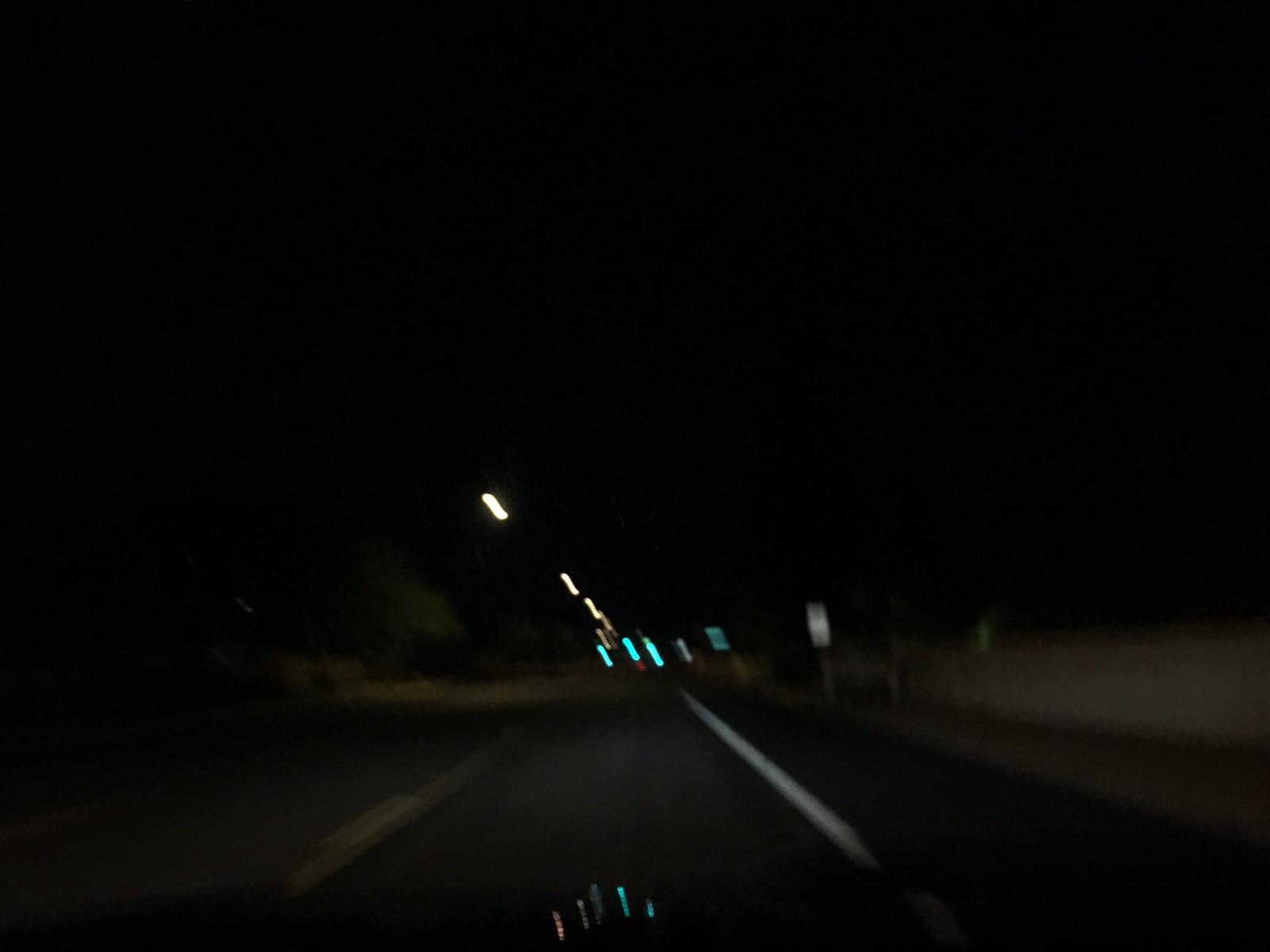The photograph captures a nighttime scene from inside a moving car, with only a small portion of the car's hood visible at the bottom. The view of the road is dominated by motion blur, creating a dynamic and slightly disorienting image. The road itself is a dark gray, flanked by a white line on the right and a yellow line on the left. Streetlights line the route, their light trails extending due to the motion, and additional green lights can be seen in the distance. A gray fence runs along the right-hand side of the road, beyond which appear blurred street signs, including white and green ones. The barely discernible outlines of trees add to the chaotic interplay of lights. The sky, occupying a large part of the background, is a solid black, accentuating the overall darkness and blurriness of the scene. The blurred light streaks, signs, and reflections contribute to an almost surreal depiction of the nighttime drive.